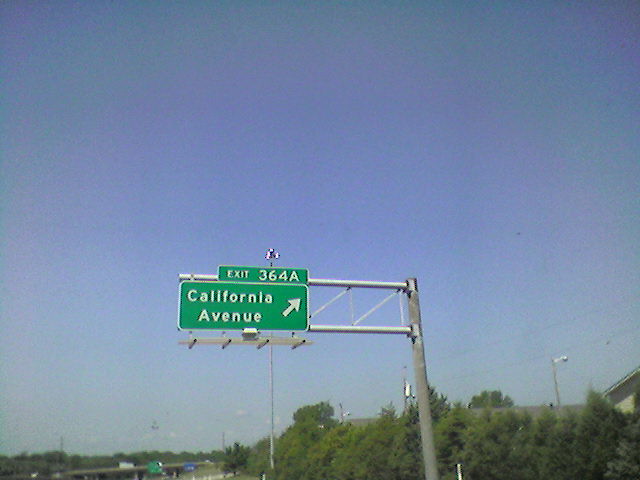A vibrant daytime photograph captures a quintessential road scene amidst clear weather. The blue sky stretches across the top of the image, adorned with faint, almost imperceptible clouds. An array of lush green trees lines the bottom, framing the snapshot of suburban tranquility. Dominating the foreground is a prominent road sign, mounted on sturdy, silver metal posts. The green and white sign directs travelers to Exit 364A, California Avenue, with an arrow pointing to the upper right, indicating the exit's direction. In the distance, an overpass is visible, accompanied by a green road sign. Street lamps and power lines are positioned behind the main road sign, adding layers of depth to the image. The photograph skillfully captures the essence of everyday road travel under a bright, clear sky.